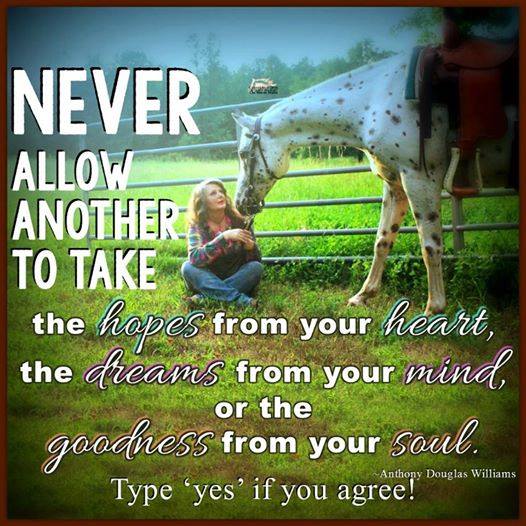In a serene, overgrown grassy pasture, a woman sits cross-legged, lovingly feeding a white horse adorned with black spots and a brown saddle. The pair is positioned beside a steel fence, under a vast blue sky with a tree line stretching across the horizon. Surrounding the tender scene is an inspiring quote by Anthony Douglas Williams, prominently displayed in large, all-caps white text on the left-hand side of the image. The quote reads, "Never allow another to take the hopes from your heart, the dreams from your mind, or the goodness from your soul." The key words—hopes, heart, dreams, mind, goodness, and soul—are elegantly highlighted in cursive outlined in green and pink. The final line encourages viewers to "Type yes if you agree."